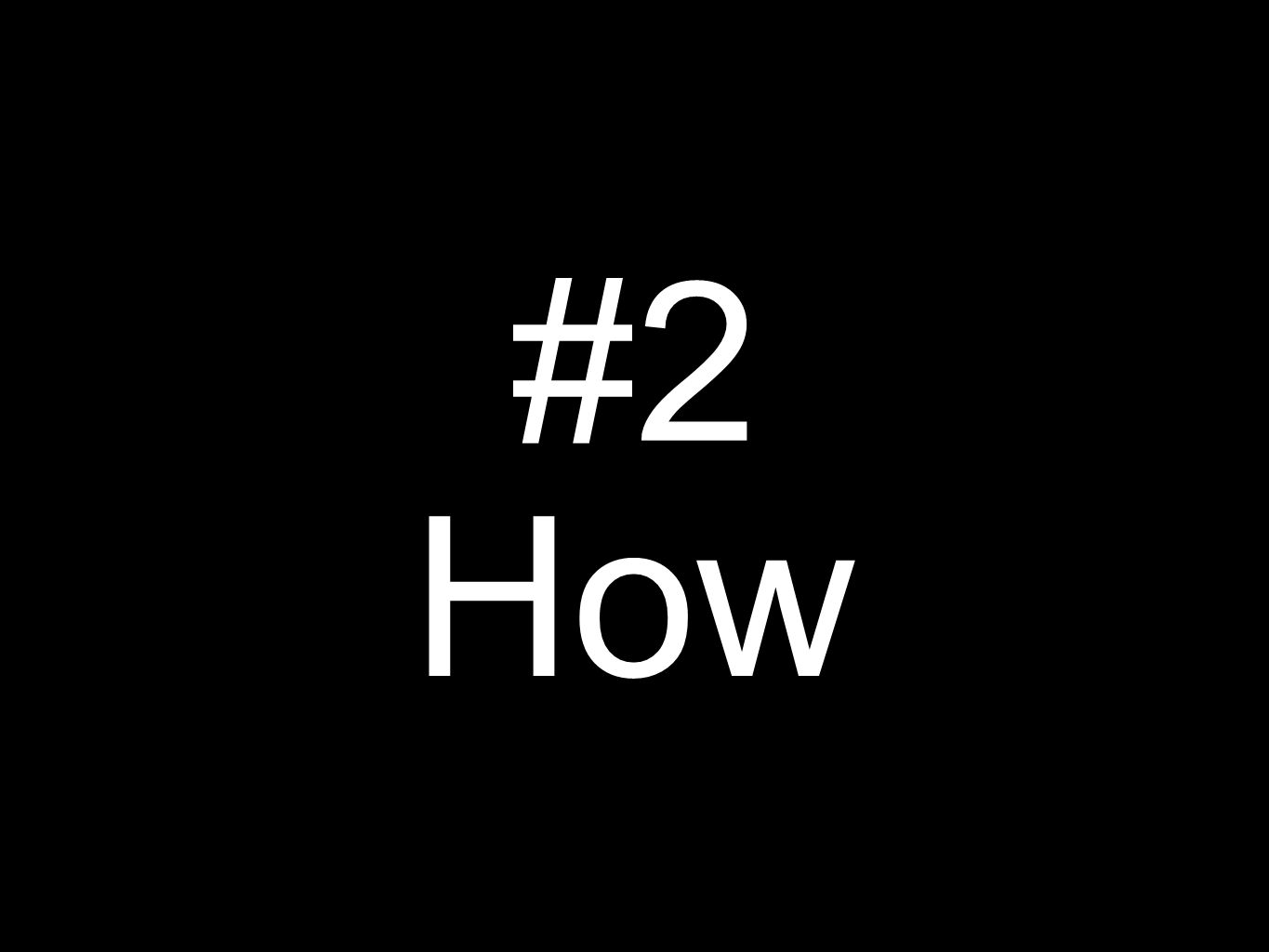The image features a completely solid black background with no objects or other elements, purely text. Centered on this dark surface are two lines of text in a very straight, large, white font. The first line displays the symbol "#" followed by the number "2." Directly below that, on the second line, is the word "HOW," with a capital 'H' and lowercase 'o' and 'w'. The stark contrast between the deep black backdrop and the clean white text catches the eye, giving the image a very bold and minimalist appearance. The positioning of the text, dead center, and its clear, large format give the impression that it might be part of a presentation slide, perhaps a title slide in a PowerPoint.